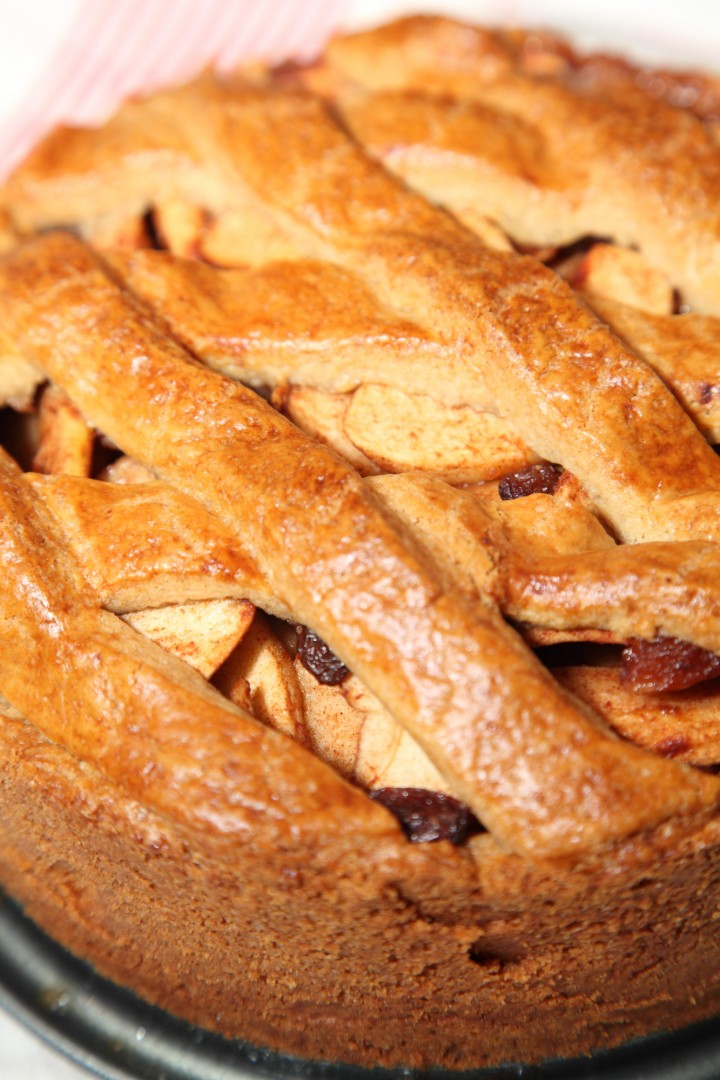The image depicts a close-up of a unique apple pie displayed on a pink and white tablecloth. The pie is presented on a gray metal serving plate and stands out with its non-traditional design. Rather than an entire pie in its shell, this pie appears cylindrical, having been cut away from its sides. The top features a beautifully woven lattice crust, glistening as though brushed with egg white before baking, revealing chunks of apples and interspersed raisins beneath. The crust is a deep, tan brown, and the overall structure has a vertical side wall approximately an inch to an inch and a half high. The lattice pattern on top is reminiscent of classic pie decoration techniques, promising a delightful, slightly crispy texture. The image captures the pie's inviting sheen and the intricate blend of its hearty filling under a well-crafted lattice crust, set against a white background that enhances its rustic charm.